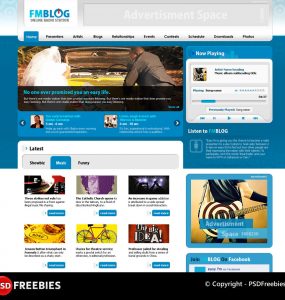The screenshot features the FM Blog, with "FM" highlighted in light blue and "Blog" in dark blue. The layout includes an advertisement space, a "Now Playing" section, and an image of a newlywed couple next to a broken-down yellow car. The bride is wearing a wedding dress, and it appears that they are attempting to fix the vehicle. There is a "Latest" section showcasing six additional images or screenshots. Towards the bottom, though slightly cut off, there is a red circle containing the white letters "SD," possibly part of a larger word. Also visible are the words "Freebies" in white and a copyright notice.